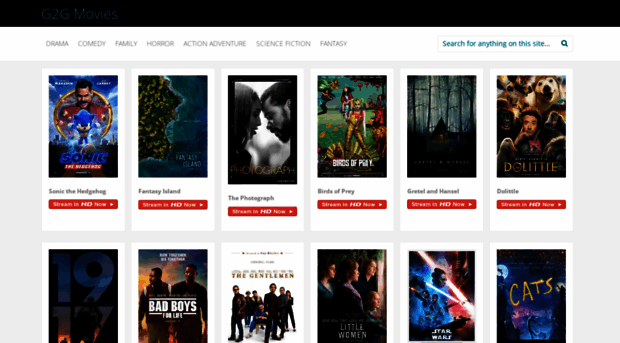The image depicts the homepage of a streaming website called "G2G Movies," designed with a clean, white and light gray background. The website features an array of clickable movie covers neatly displayed in a grid format. Some of the movies highlighted include recent releases such as "Sonic the Hedgehog," "Fantasy Island," "Birds of Prey," "Doolittle," "Bad Boys for Life," "1917," "Little Women," "Star Wars: The Rise of Skywalker," and "Cats." Each movie cover has a corresponding "Stream in HD Now" button below it.

At the top of the page, there is a search bar located on the right side, allowing users to find specific movies quickly. On the left side, there are genre selection options, including drama, comedy, family, horror, action, adventure, science fiction, and fantasy, facilitating easy navigation through various types of films. The inclusion of newly released titles such as "Bad Boys for Life," suggests that the screenshot is relatively recent. The movie selection, predominantly consisting of contemporary films, lacks classic titles, indicating that the website is focused on more recent content.